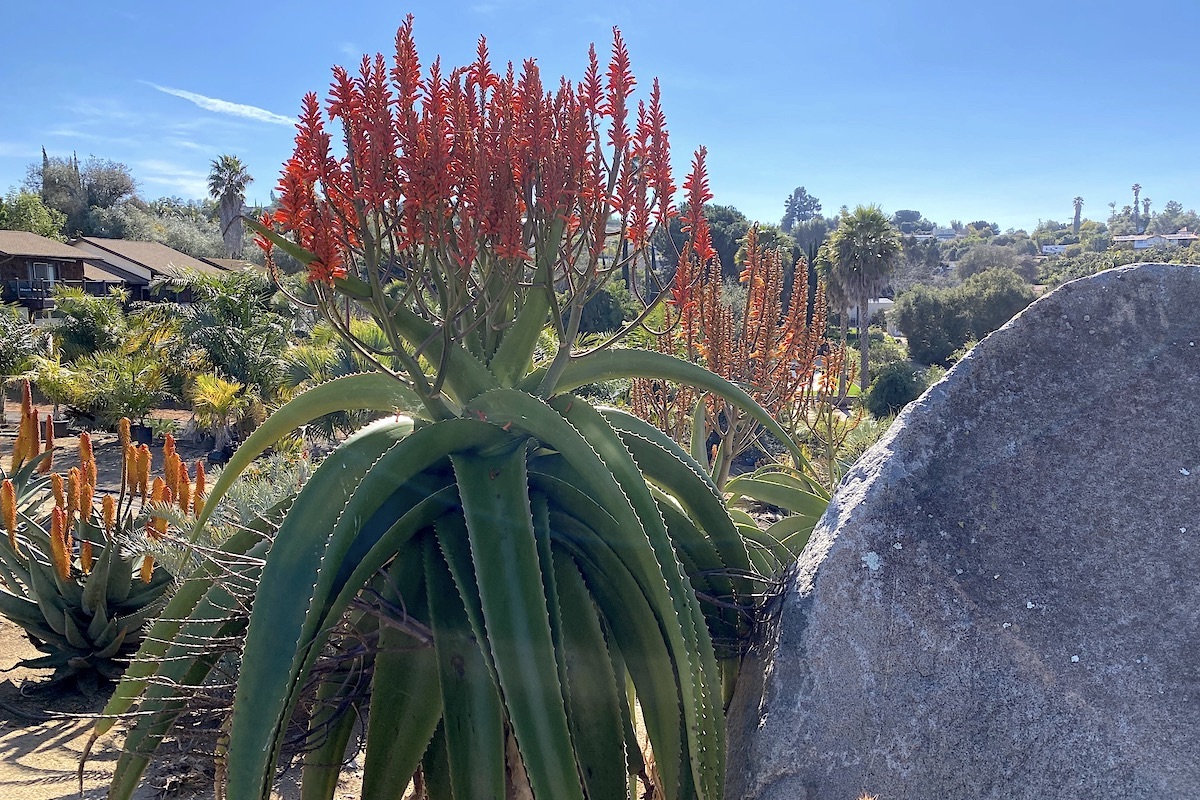This image captures a striking desert landscape with a central focus on a large, lush cactus plant. The plant, resembling an aloe vera with its numerous green, elongated leaves curving gracefully toward the ground, dominates the center of the photo. These leaves form about three or four overlapping layers, each edged with tiny, white prickly spikes. Towering from the center of the plant are approximately two to three dozen orange, cone-shaped flowers on gray stems, all pointing skyward, giving a vibrant contrast against the deep blue, clear sky.

To the right of the cactus, a substantial, flat-surfaced gray rock with a curved top catches the sunlight, adding a textural element to the scene. In the background, two additional, shorter cacti of different species are visible. One to the left and another behind the main cactus, also flaunting green leaves and orange flowers. Surrounding these primary plants are various desert shrubs, complemented by the distant silhouette of green palm trees and a house peeking from the upper left corner, completing this picturesque desert view.